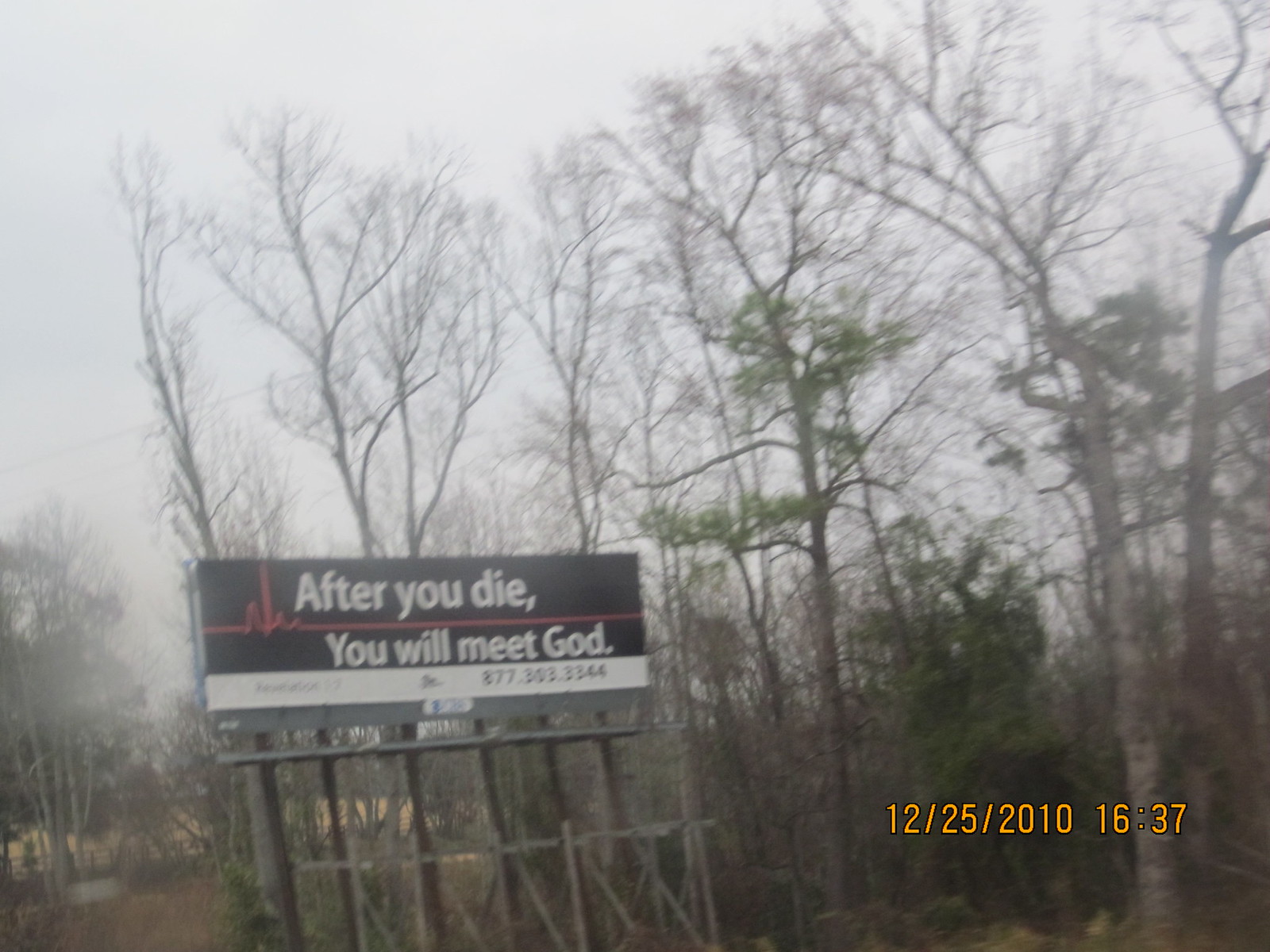In this outdoor winter photograph, a prominent black billboard stands amidst a backdrop of mostly bare trees under a gray, cloudy sky. One tree has a few remaining leaves, contrasting with the other barren branches. The ground is earthy with no visible snow. The imposing billboard carries a solemn message in white text, flanked by a red lifeline graphic reminiscent of a hospital monitor's heartbeat. It declares, "After you die, you will meet God." Beneath this, in a slightly blurred section, a phone number appears: possibly 877-303-8344. Wooden scaffolding supports the billboard, which dominates the scene. In the lower right corner of the image, an orange timestamp reads "12/25/2010 16:37," marking the date and time this moment was captured. No vehicles are visible, further emphasizing the desolate, wintry atmosphere of the wooded area.